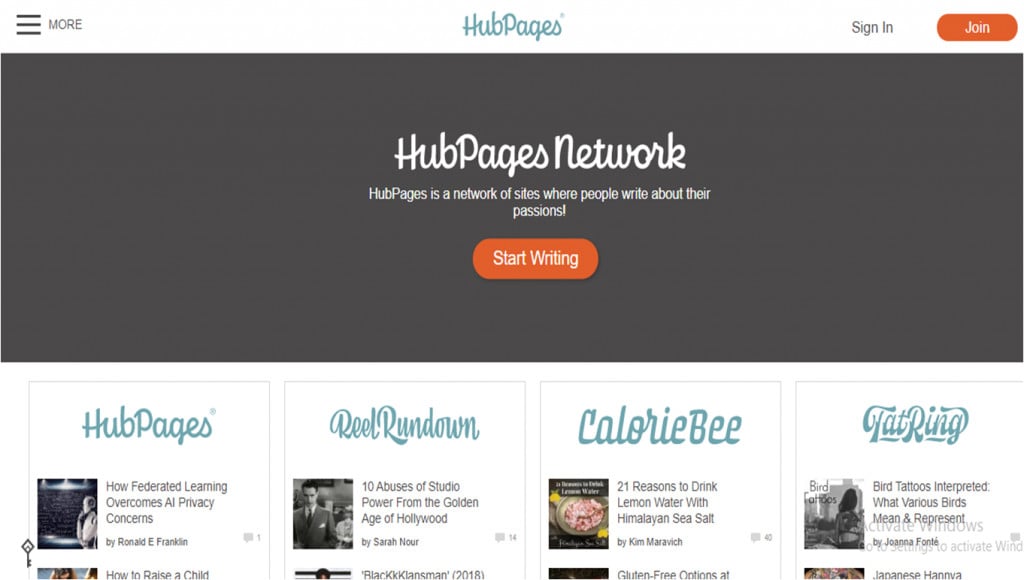The image depicts a screenshot of the Hub Pages Network website. In the top-left corner, there is a "More" menu that can be expanded to reveal various options. At the center top, the website's name and logo, "Hub Pages," are prominently displayed in blue. To the right of the logo are two buttons: a "Sign In" button and an orange "Join" button. 

The centerpiece of the website features a grey panel with an informative caption in large white font: "Hub Pages Network." Below this, in smaller white font, is a description stating that Hub Pages is a network of sites where people write about their passions. An orange button labeled "Start Writing" is placed centrally below this text.

Beneath the grey panel are four white tiles, each bordered by a thin grey line. The first tile, titled "Hub Pages" in blue, addresses how federated learning overcomes privacy concerns. The second tile, titled "Real Rundown," presents an article about "10 Abuses of Studio Power from the Golden Age of Hollywood." The third tile, named "Calorie B," discusses "21 Reasons to Drink Lemon Water with Himalayan Sea Salt." The fourth tile, titled "Tat Ring," explores bird tattoos, explaining what various birds symbolize and represent.